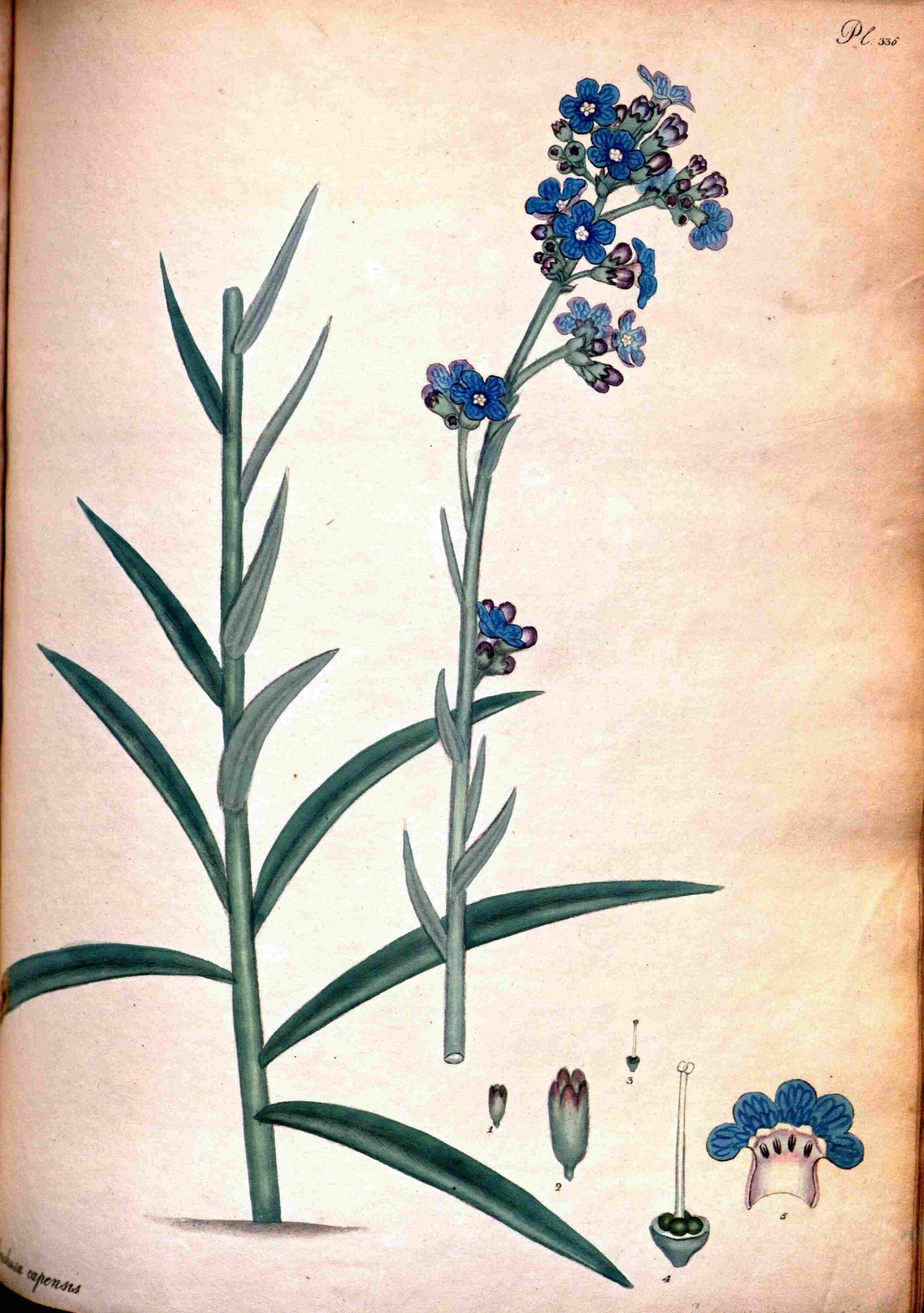The image portrays a detailed botanical illustration on what appears to be a beige parchment or scroll, likely a sketch or watercolor from the 18th or 19th century. On the left side, there is a tall, dark green plant with long spear-like leaves, depicted without any flowers. This contrasts with the central focus of the image: a striking stalk adorned with numerous small, vibrant blue flowers clustered at the top. The flower’s stem is long and light green. 

In the bottom right, the illustration transitions into a diagram-like format, showcasing the different parts of the plant, each meticulously detailed and numbered from 1 to 5, highlighting the various layers and structures of the flower. The top right corner of the parchment features a signature by the artist, providing an authentic touch. Additionally, there is some small, barely legible text on the bottom left of the parchment, contributing to the illustration's antiquated and scholarly feel. This composition enriches the image, making it an exquisite blend of art and science, ideal for a botany book.